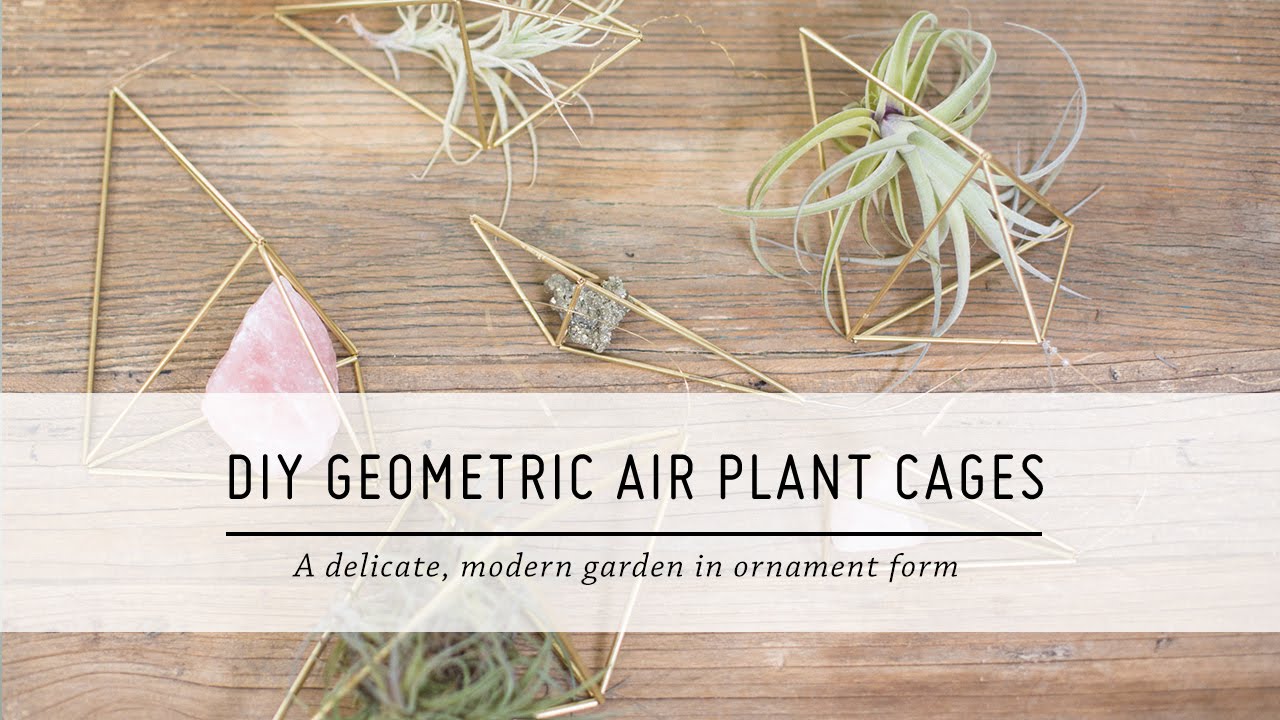In the photograph, we see an advertisement for DIY Geometric Airplant Cages. The emphasis is on a delicate, modern garden presented in ornamental form. The geometric shapes, made from thin brass or bronze tubes, resemble pyramidal structures or small collections of interconnected triangles, creating variously sized interior spaces.

The scene is set on a light-stained wooden table composed of multiple connected boards. Five geometric structures are arranged on this table. Three of these structures house air plants, characterized by their light root systems and gracefully curved, green fronds resembling succulents. The remaining two structures contain stones or crystals, with one stone appearing pink and another greenish-gray.

Across the page, the text reads "Do-It-Yourself DIY Geometric Airplant Cages," with a smaller print describing the product as "a delicate modern garden in ornament form." The overall arrangement highlights both the elegant, minimalistic design of the geometric planters and the unique combination of natural elements they encase.